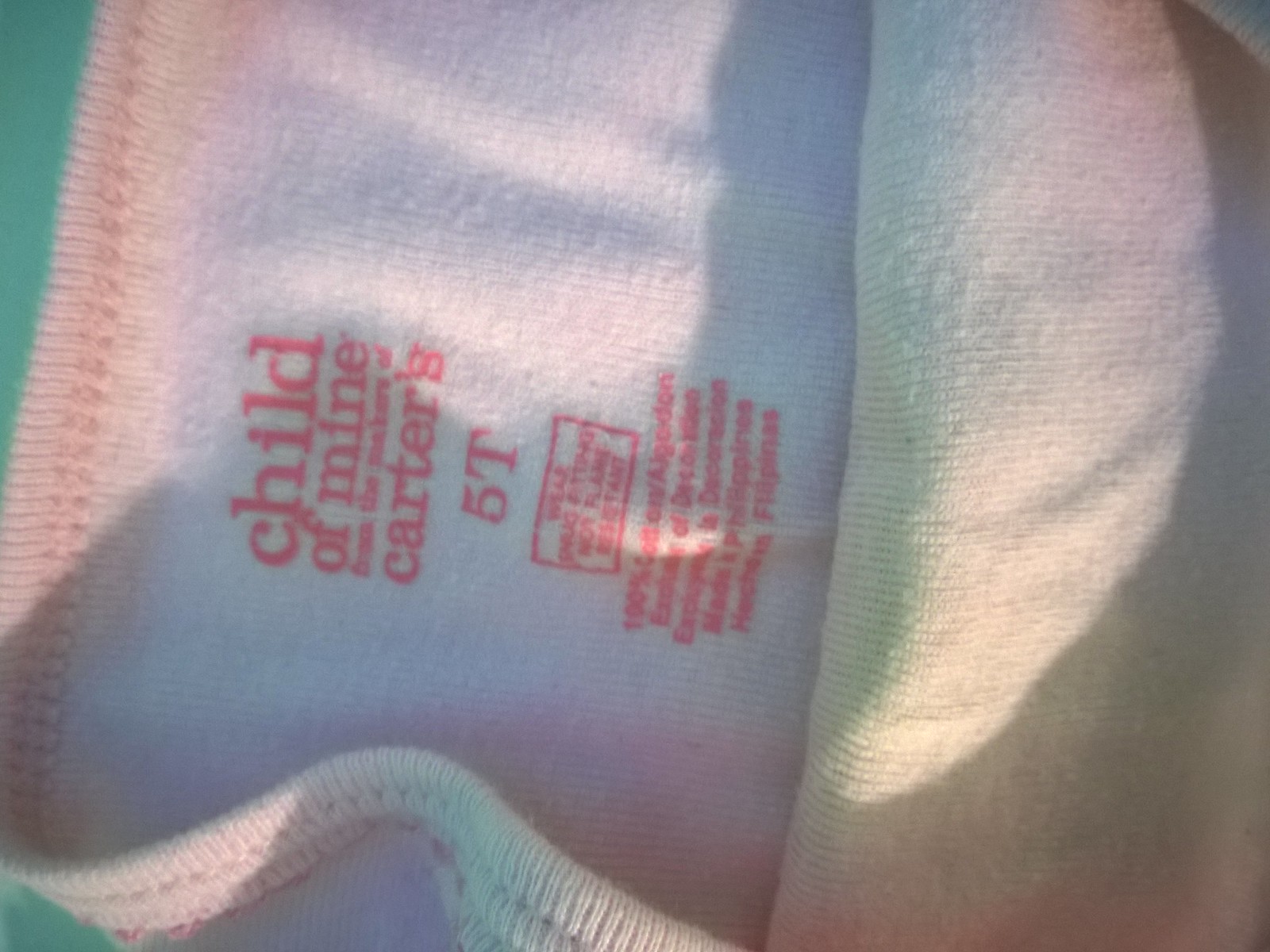This photograph is a close-up of the inside tag area of a piece of children's clothing, specifically turned so that the top of the clothing is to the left. The material appears to be white cotton, although the lighting causes parts of it to look light purple, light pink, light green, or even yellow. The tag text, printed in red or pink letters, reads "Child of Mine from the Makers of Carter's" and designates the size as 5T. There is a rectangular section with more writing in red, which is difficult to decipher. Below this, it states "100% cotton." Underneath, faded and hard-to-read text is present. The upper and right portions of the image are illuminated by a patch of sunlight, while a shadow cast over the left side makes that part look dark gray. The fabric features an embroidered collar in a bright, almost fluorescent green.